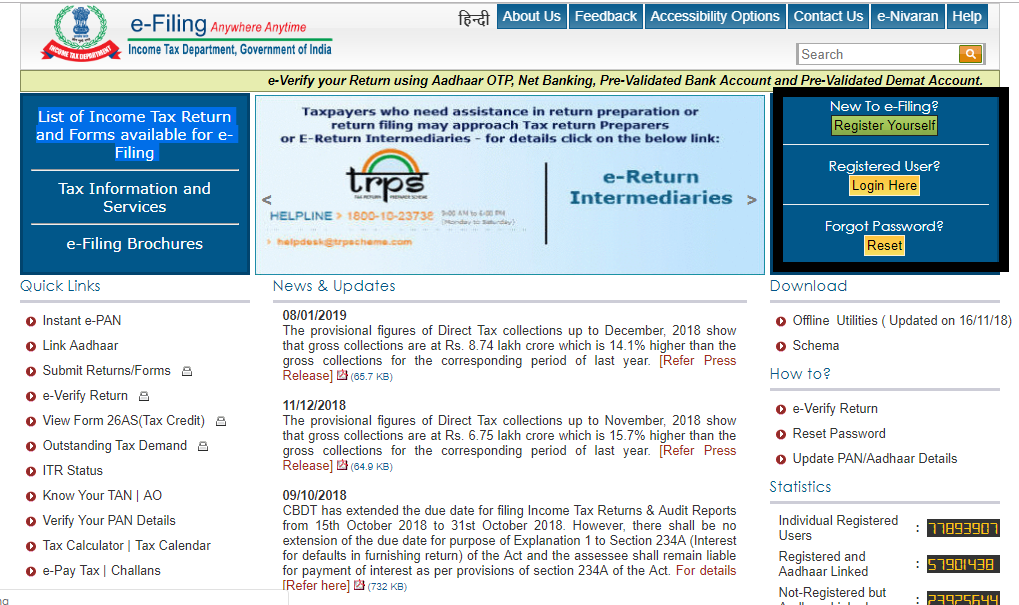This screenshot captures an intricate webpage, brimming with information and resources primarily related to e-filing tax returns. Dominating the top of the page are bold banners with slogans such as "e-Filing: Anywhere, Anytime," setting an inviting tone. The website provides a comprehensive catalog titled "List of Income Tax Return and Forms Available for e-Filing," clearly indicating its utility.

A prominent section labeled "Tax Information and Services" features a variety of resources, including e-filing brochures. The left sidebar is adorned with a multitude of quick links that facilitate user access to essential tools and forms, such as "Instant E-PAN," "Link Aadhaar," and "Submit Return Forms." Additional functionalities listed in this sidebar include "E-Verify Return," "View Form," and several others, like "Outstanding Tax Demand," "ITR Status," "Know Your TAN/AO," "Verify Your PAN Details," "Tax Calculator," and a dedicated "E-Pay Tax" area towards the bottom.

The upper portion of the page showcases a section defined by the acronym "TRPS," embellished with a colorful rainbow backdrop, possibly indicating a specialized program or service. Additionally, there is a highlighted area titled "E-Return Intermediary," further guiding users through their e-filing journey. The overall layout is methodically arranged, designed to provide ease of navigation through its multifaceted offerings.